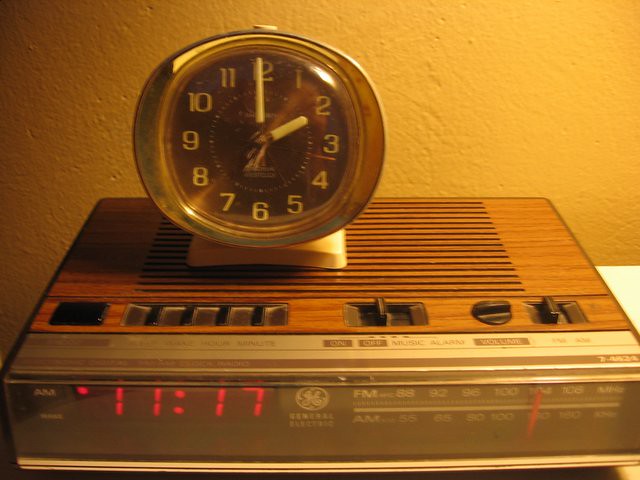This image features a vintage setup with two clocks, reflecting a nostalgic aura reminiscent of the 1970s or 1980s. At the forefront is a classic analog clock, highlighted by its sleek silver or metallic border. Against a stark black background, the white numerals and matching hour and minute hands stand out prominently. The analog clock, displaying a time around 2 o'clock, sits gracefully atop a retro digital clock radio.

The digital clock radio, likely from General Electric, exudes vintage charm with its faux brown wood plastic finish covering the speaker section. The black dials adjacent to it control volume and alarm settings, providing functional and aesthetic appeal. The digital display shows the current time as 11:17 a.m. Meanwhile, the radio tuner, marked by a distinct red dial, is precisely set at 104 FM, denoted in white text, indicating a station is tuned in. This photograph beautifully captures the juxtaposition of analog and digital elements from a bygone era.